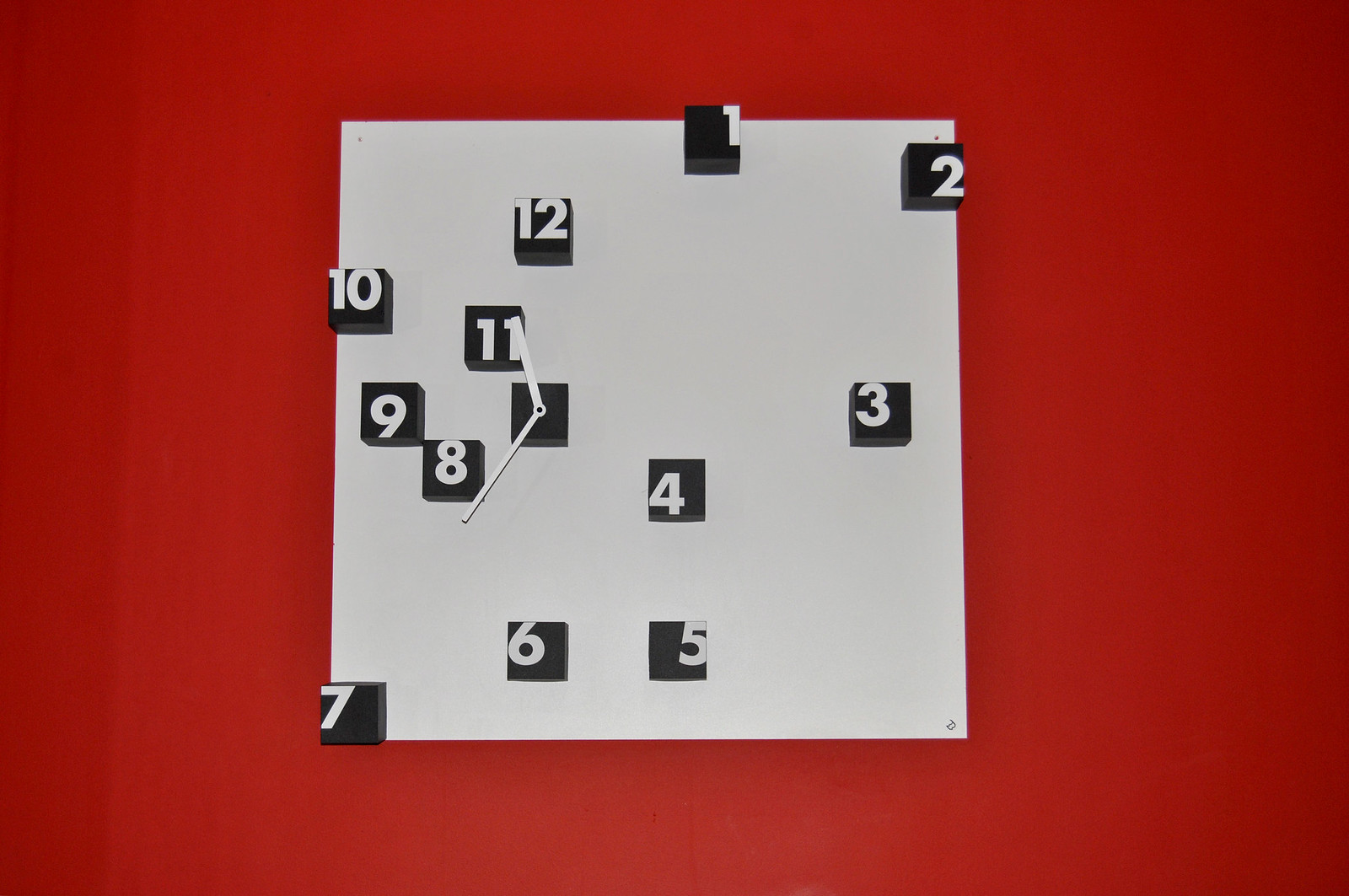The image features a red background with a medium gray square prominently centered. Scattered across the gray square are black squares inscribed with white numbers ranging from 1 to 12, randomly distributed and occasionally overlapping the edges of the gray area. None of these numbers are centered within their squares. On the left side of the gray square, there is another black square containing white clock hands—the hour hand pointing to the top and the minute hand extending to the bottom left, indicating the time is approximately 11:35. Additionally, there is a small symbol located at the bottom right of the gray square. This composition resembles an abstract, modern art version of a clock.